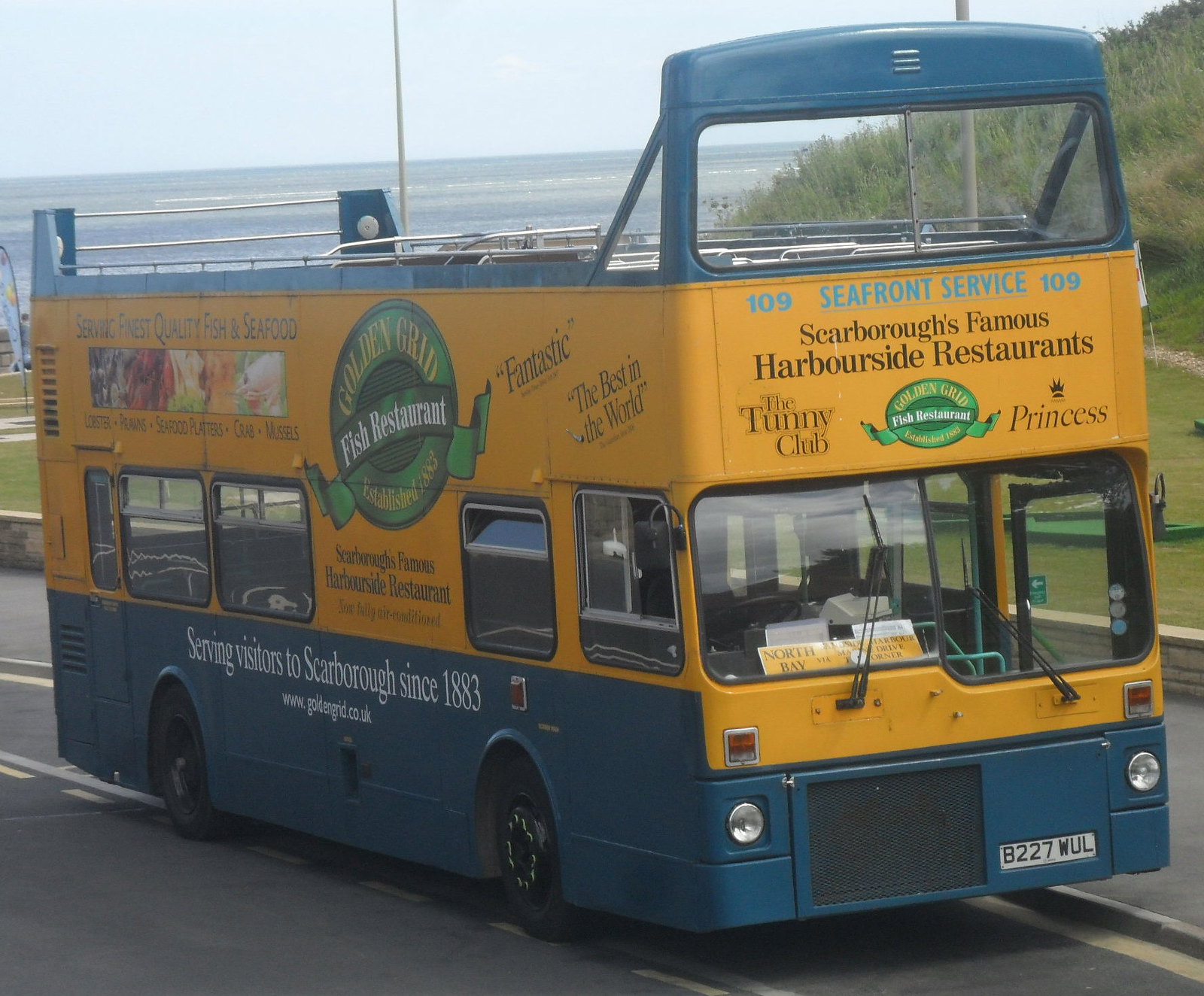The image is a detailed photograph of a double-decker tour bus in motion, facing slightly towards the camera to the right, and traveling down a gray paved street near the curb. The bus has distinctive coloration: the bottom part and the top rim are a medium blue-green, while the entire middle section is a bright golden yellow. It features an open top, allowing passengers to view the surrounding area.

Prominent advertisements and text are visible on the bus. The front section displays the route number "109 Seafront Service" and the message "Scarborough's Famous Harborside Restaurants." The name "Golden Grid Fish Restaurant" appears in a green oval logo on the side, with phrases like "Fantastic" and "The best in the world" scattered around it. Additional text, "Serving visitors to Scarborough since 1883," is printed in white at the bottom, and there's likely a web address below it, although it's unreadable.

The background shows a hint of a light blue ocean to the left and a grassy hill ascending on the right, under a very light blue hazy sky, emphasizing the bus's coastal route and scenic surroundings.